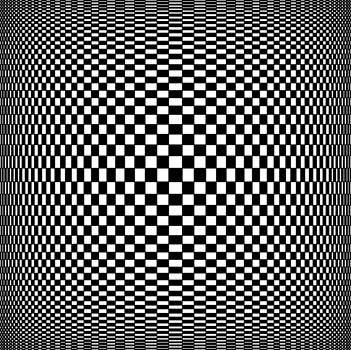The image is a black and white abstract square pattern evoking a retro 70s vibe. At its core, larger squares form what appears to be a circle. As the pattern radiates outward, the squares become progressively smaller, creating an optical illusion that can look three-dimensional. This central circle transitions into a triangular form at the corners where the squares continue to shrink. Horizontally, the squares widen yet remain short, while vertically, they become taller but more slender. This geometrical design, composed entirely of squares, seems to morph and almost dissolve at the edges due to the minimal spacing, enhancing its intricate checkerboard effect.